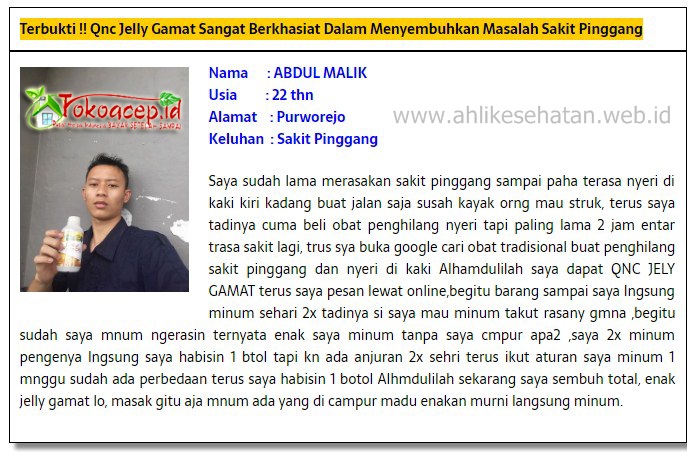The image appears to be a screenshot of an informational ID card, primarily written in a foreign language. The card has a white background with multiple sections of text, some of which are highlighted in yellow. At the top, there is a name "Abdul Malik" with an age field likely denoted as "USIA 22THN" indicating the person is 22 years old. The card includes an address field labeled "Alamat, Pavorajo, PURWOREJO" and a medical condition or note "Caluhan, KELUHAN, Sakit Pingang." There is a black paragraph of text providing a short biography of Abdul Malik. 

A young man with short brown to black hair is depicted on the left side of the image. He is wearing a navy or black polo shirt and holding a drink. Above him is a logo that reads "Toko Asep.id" featuring a house with a green roof. Another website, "www.ahlikesehatan.web.id," is mentioned in the grey text. The layout includes blue and black writing, with the text on top also highlighted in yellow. Overall, the card provides personal and medical details about Abdul Malik, complete with an ID photo and web addresses.